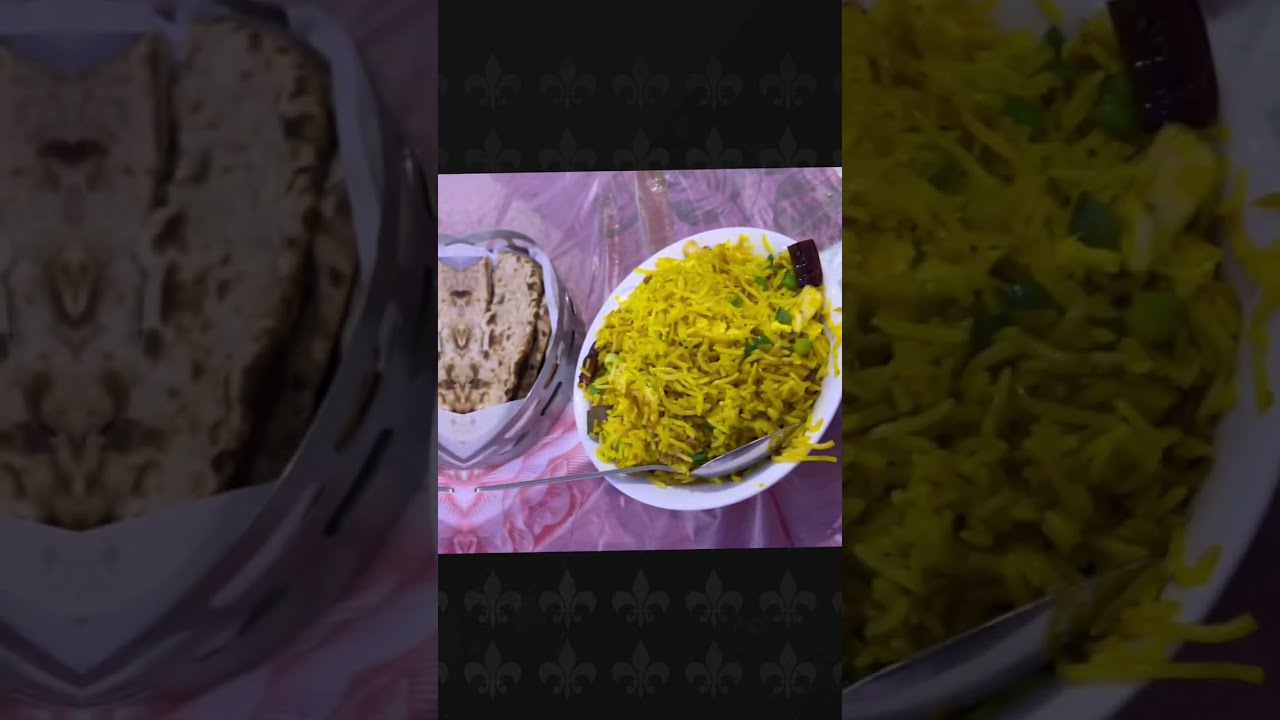The main image in the center panel features a white bowl of yellow noodles, possibly ramen, accompanied by various vegetables and a spoon. To the right of the bowl, on what appears to be a metallic or heart-shaped plate, there is a serving of light brown meat, potentially resembling hamburger patties. The entire setup is placed on a table with a light pink, possibly white and pink tablecloth. The left and right thirds of the whole image comprise blurred, blown-up sections of the central image; the left highlights the meat portion, while the right focuses on the bowl of noodles. Surrounding the central image, there are faint gray panels. Additionally, faint symbols like fleurs-de-lis can be discerned within some of the darker rectangles framing the central image. The dominant colors in the scene include yellow from the noodles, white from the bowl, pink from the tablecloth, and hints of gray and silver.